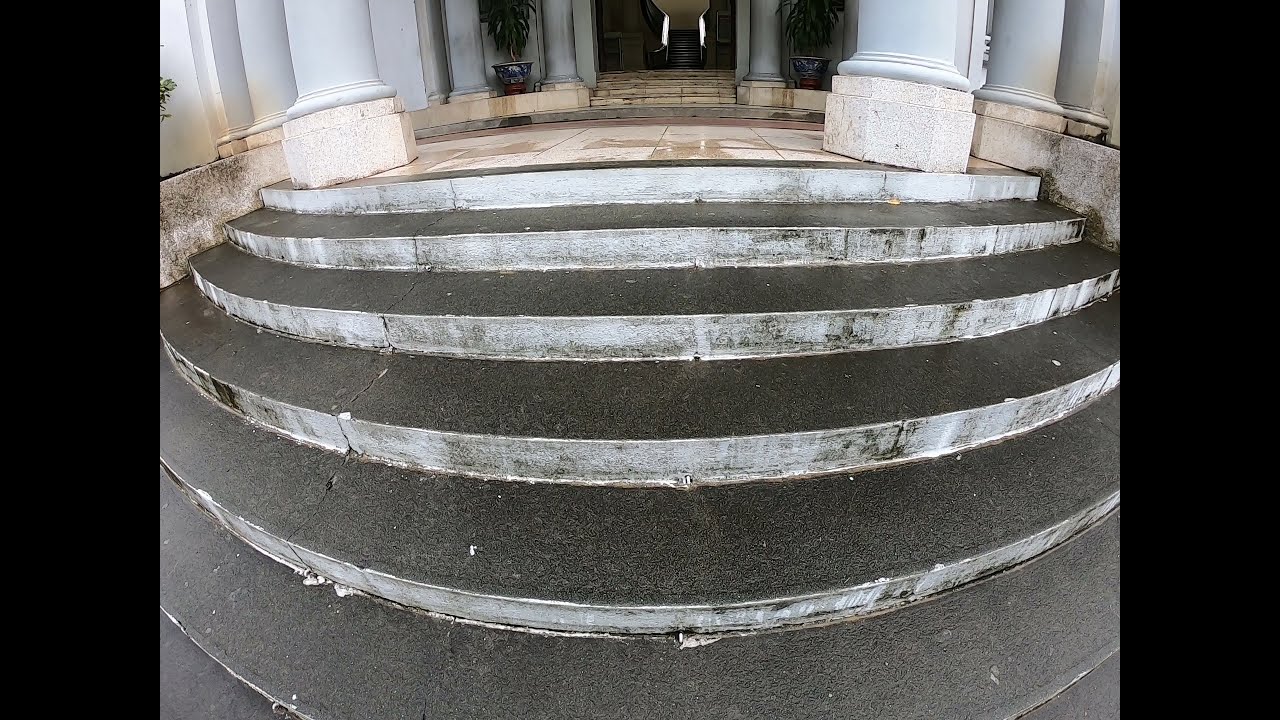This image captures the entrance of an old, possibly governmental or upscale building, characterized by a series of black stone steps leading upward. There are six prominent steps in the foreground, suggesting the start of a primary staircase. The steps guide the viewer to a landing area, flanked by two white pillars, which then leads to more steps ascending into the building. This entrance area is decorated with large, peach-colored tiles, adding a distinct aesthetic to the porch.

On either side of the entryway, there are two identical potted plants housed in large, blue and white porcelain vases. The tropical plants have lush green leaves, contributing to the inviting atmosphere of the entrance. Despite the architectural details, including the thick concrete steps and the white pillars, the image does not reveal much of the building itself, focusing instead on the entrance and stairway. No people are visible in the scene, emphasizing the still and empty nature of the setting.